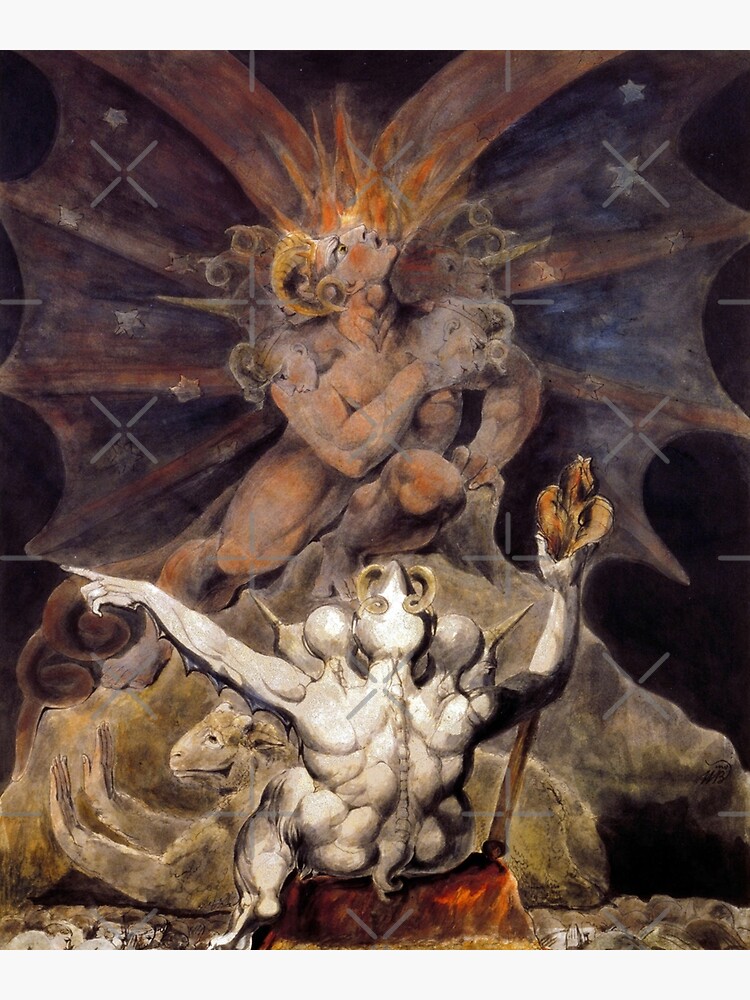The image depicts a mythological scene reminiscent of William Blake's style, featuring intricate and fantastical elements. At the center stands a striking figure with a large, ornately designed wingspan, colored in tans, reds, oranges, and creams. This figure, reddish-brown with horns on its head, gazes upwards. Draped over the figure's shoulders is another person, adding to the surreal composition. Facing them is a peculiar white creature, viewed from the back, with three heads and an arm extended outward while the other clutches a rod-like staff or sword. Below, a bizarre lamb-like animal with human hands lies on the ground. The overall ambiance of the image is eerie and otherworldly, enriched by its vivid details and mythological essence.